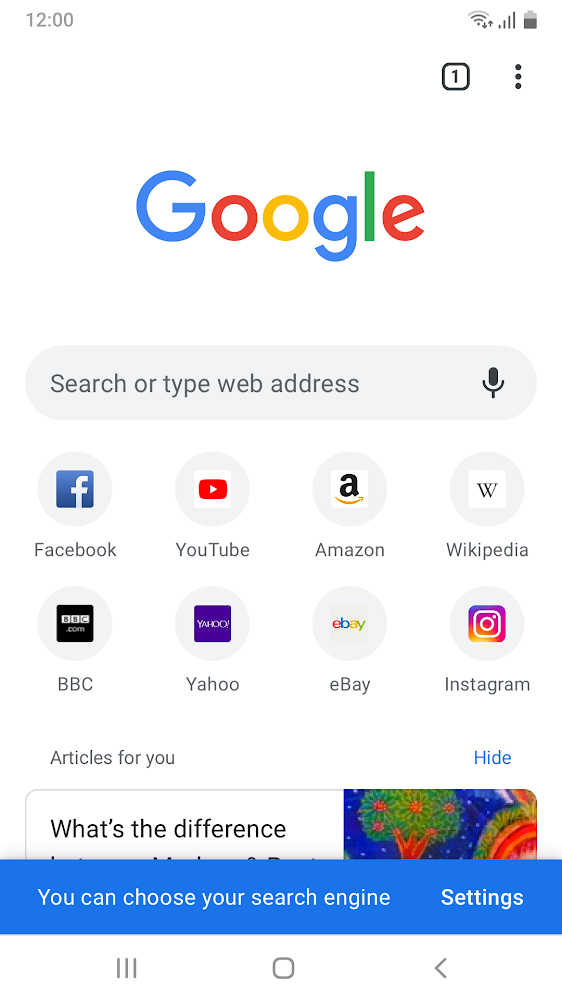The screenshot captures a cell phone's home screen, precisely at 12 o'clock, as indicated by the top bar alongside the icons for Wi-Fi connectivity, signal coverage, and battery life. Dominating the middle is the familiar "Google" logo, displayed in its iconic sequence of blue, red, yellow, blue, green, and red letters, above a search bar prompting "Search or type web address."

Below the search bar, a series of app icons are neatly arranged in a grid format:
- **Facebook:** Represented by a blue square featuring a lowercase 'f' in white at the lower right side.
- **YouTube:** Displayed within a white square containing a red rectangle with a white play arrow in the center.
- **Amazon:** Identified by a white square with a black lowercase 'a', accompanied by an underlining curve that suggests a smile.
- **Wikipedia:** Enclosed in a white square, showcasing a black uppercase 'W' in the middle.
- **BBC:** Shown as a black square with three smaller adjoining white squares that spell out "BBC".
- **Yahoo:** Marked by a purple square inscribed with "Yahoo" in white letters.
- **eBay:** Illustrated by a white square with "eBay" in lowercase, multi-colored letters of red, blue, yellow, and green.
- **Instagram:** Noted by a gradient square of purple, orange, and red hues, centered with a white camera icon.

Beneath these icons, the interface includes a section titled "Articles for you," offering personalized content. At the very bottom, partially cut off, the text indicates additional options, stating, "You can choose your search engine settings."